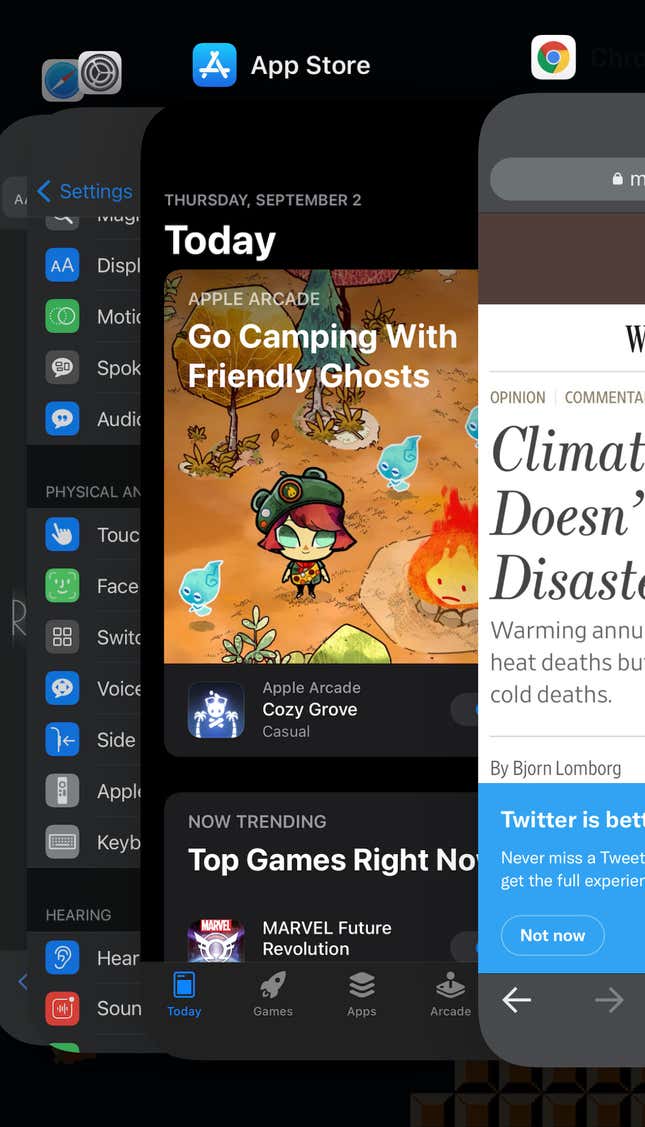The image appears to be a screenshot of an iPhone showcasing the currently open apps. Four apps are displayed:

1. **Google Chrome (Right)**: Google Chrome is open to an article about climate change and natural disasters, although the text is cut off making it difficult to read the full content. Below the article, there is a Twitter advertisement suggesting creating or opening a Twitter account.

2. **App Store (Middle)**: The App Store app is highlighting a feature for "Apple Arcade." The first item on the page is dated "Thursday, September 12th," followed by "Today" in bold white text. An advertisement for the game "Cozy Grove" is prominently displayed, showing an image with four ghost sprites and a ghost campfire. The text underneath reads, "Apple Arcade - Go camping with friendly goats," and describes the game as "casual." Below this, trending games are showcased, with "Marvel Future Revolution" being one of them.

3. **Settings (Left)**: The Settings app is open, showing various options like display, motion, and audio. The interface is in dark mode, presenting a sleek black, white, and gray aesthetic typical of modern smartphone settings.

4. **Safari (Far Left)**: Tucked away behind the Settings app, the Safari icon is also visible, conforming to the dark mode theme.

The overall interface is characterized by its modern, sleek design, with a predominant use of dark mode to minimize bright colors, enhancing readability and user comfort.